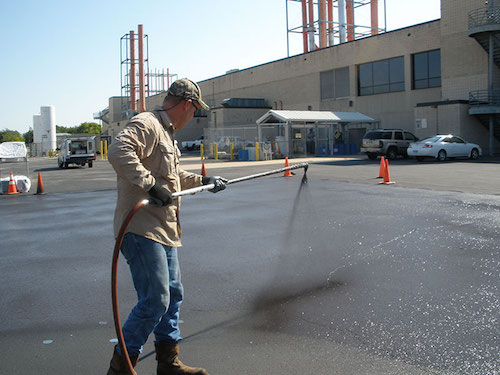A man wearing a beige jacket, blue jeans, brown boots, a baseball cap, and black gloves is power washing or applying a spray substance onto a paved parking lot. He is using a wand connected to a hose, directing the stream downwards towards the ground. The scene is set outdoors during the daytime, with a bright blue sky overhead providing natural light. The background features a long, wide, beige-colored building resembling a professional business or warehouse, with several vehicles parked in front. Orange traffic cones are placed around the area where the man is working. Further in the distance, large green trees and a couple of white storage tanks can be seen, possibly indicating a chemical plant or industrial setting. The entire image has a clear, detailed, and representational style, capturing the essence of a workday task in an industrial parking lot.